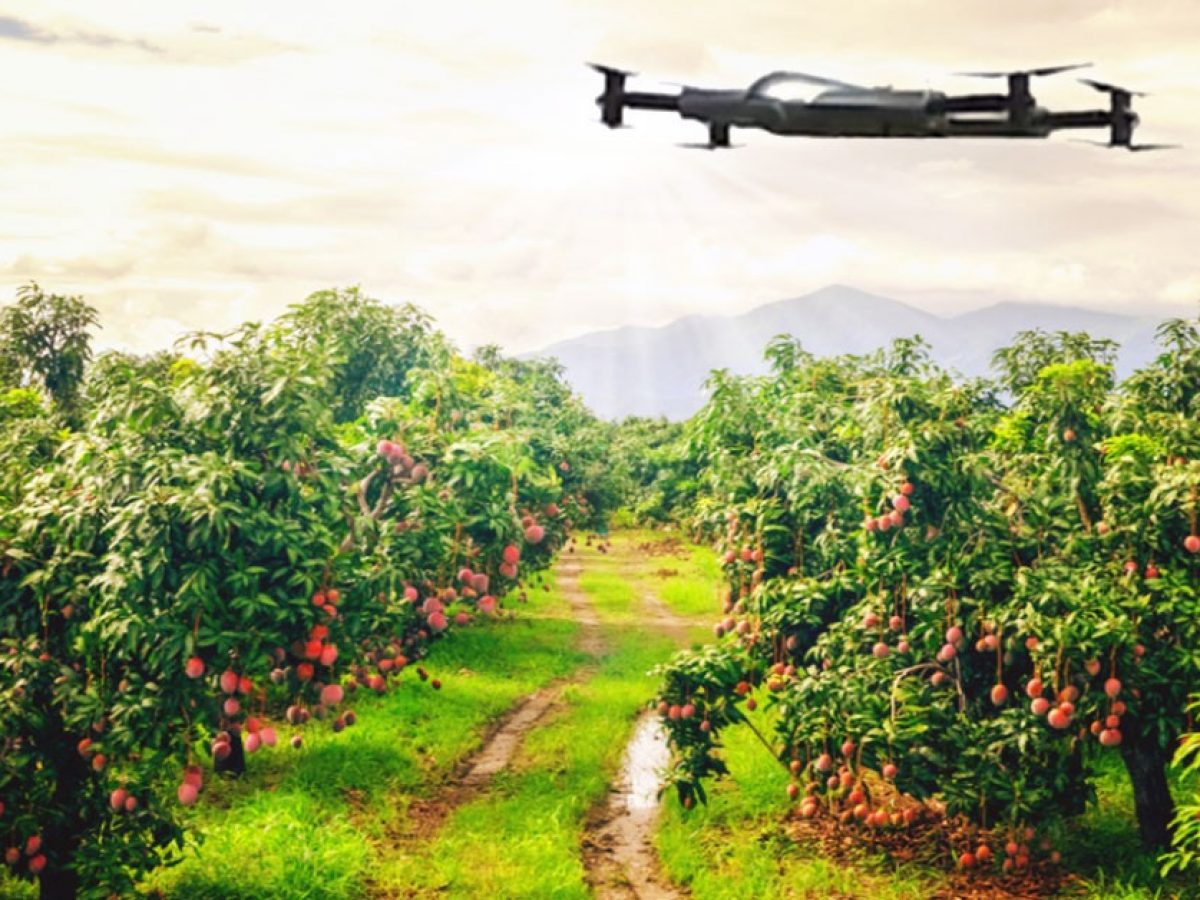The image depicts a sprawling orchard with rows of green trees that have tire-marked mud tracks running between them, indicating frequent vehicle passage. These tracks have indented the grassy path, suggesting wet ground. The trees are dense with vibrant green leaves and bear reddish to purplish, roughly apple-sized fruits, some of which appear to be on the ground hinting at minor damage. The fruits hang delicately, contrasting with the dark bark of the trees. The sky above is partly cloudy with sunbeams filtering through, casting a warm light over the orchard. A black drone equipped with four propellers hovers in the upper right portion of the image, slightly to the side yet significant. In the distance, faint outlines of a mountain range complete the picturesque scene.